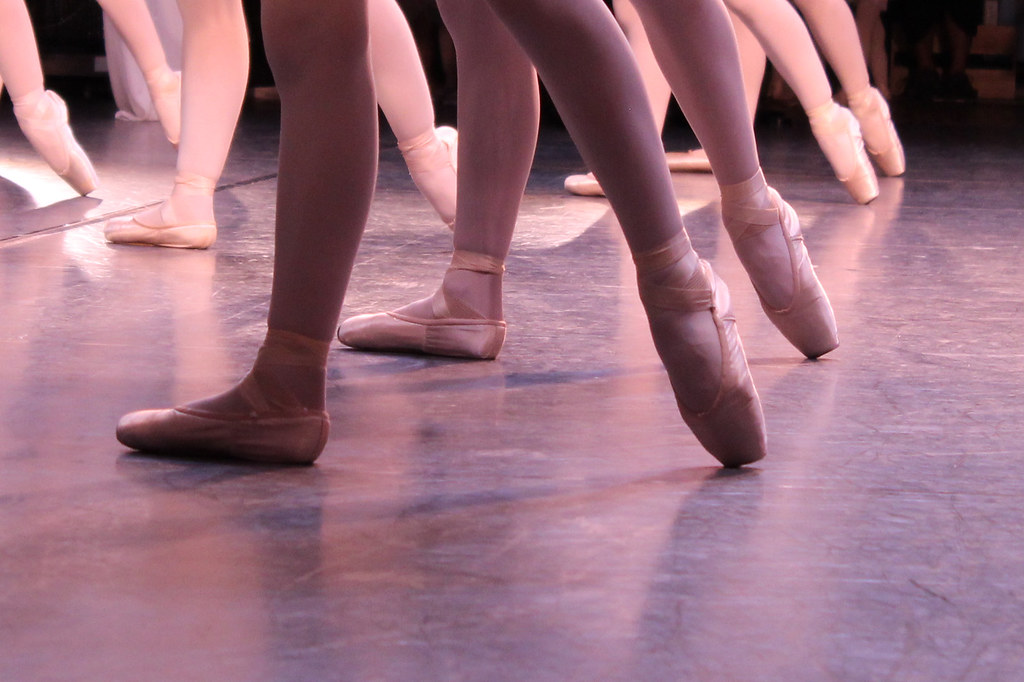This photograph captures a ballet practice session in a dance studio, focusing on the lower legs of the dancers. Prominently featured are five pairs of legs, totaling ten legs, arranged with four pairs standing together in a line and one pair near the left side, adjacent to a mirror reflecting two legs. The dancers are positioned with one foot flat on the floor and the other foot pointed, touching the dance floor with satin ballet slippers in light peach or light pink. The image reveals the wear and tear typical of ballet practice, as the repetitive strain of dancing has visibly damaged some of the feet. The dancers are practicing on what appears to be a smooth, possibly marble or stone floor, under soft lighting, further emphasizing the pastel hues of their attire. In the dimly lit background, faint outlines of additional legs can be discerned, adding depth to the scene. Though the image lacks any text or identifying markers, the dedication and discipline of the ballerinas are evident.